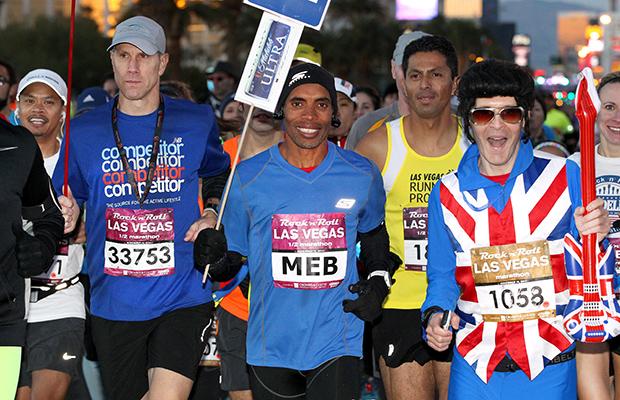The photograph captures a bustling athletic event, presumably a marathon, held in Las Vegas with the banner "Rock and Roll Las Vegas" prominently displayed on the bibs of the participants. Dominating the foreground are four runners who occupy about 90% of the frame. The man on the far right stands out in a colorful Union Jack vest, holding an inflatable guitar with the same pattern, and wearing dark sunglasses. Next to him, a runner in a yellow tank top contrasts against the backdrop. The third man from the right, dressed warmly in a blue shirt, gloves, and a hat, holds a sign advertising a beer company. The fourth highlighted runner, also in a blue shirt and a gray hat, holds another partially visible sign. Behind these central figures, a sea of marathon participants stretches into the background, progressively blurring into what appears to be a cityscape, with many runners looking happy and directly at the camera. The mix of athletic attire and signage, along with the variety in the runners' expressions, vividly conveys the energetic atmosphere of the event.